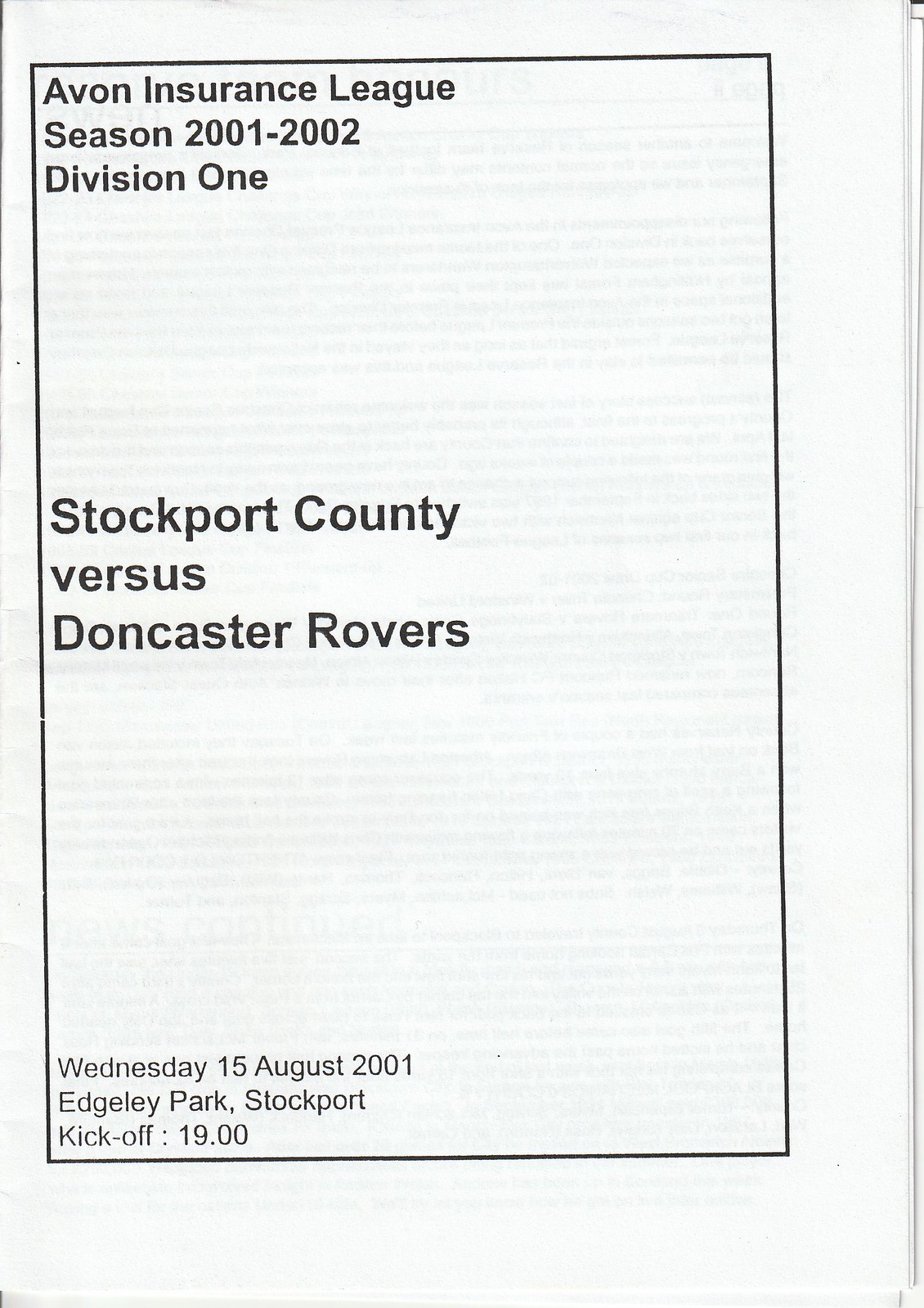The image showcases a somewhat aged soccer program from the Avon Insurance League, Season 2001-2002, Division 1. The white paper, framed by a thin black rectangle, features black text that stands out clearly. In the upper left corner, it reads "Avon Insurance League" followed by "Season 2001-2002" and "Division 1." The central portion of the page prominently displays "Stockport County versus Doncaster Rovers." At the bottom left, the details of the match are given: "Wednesday 15 August 2001, Edgeley Park, Stockport, kickoff 1900." The paper appears slightly see-through, hinting at some indistinct background text, and the program indicates it's from over 20 years ago.